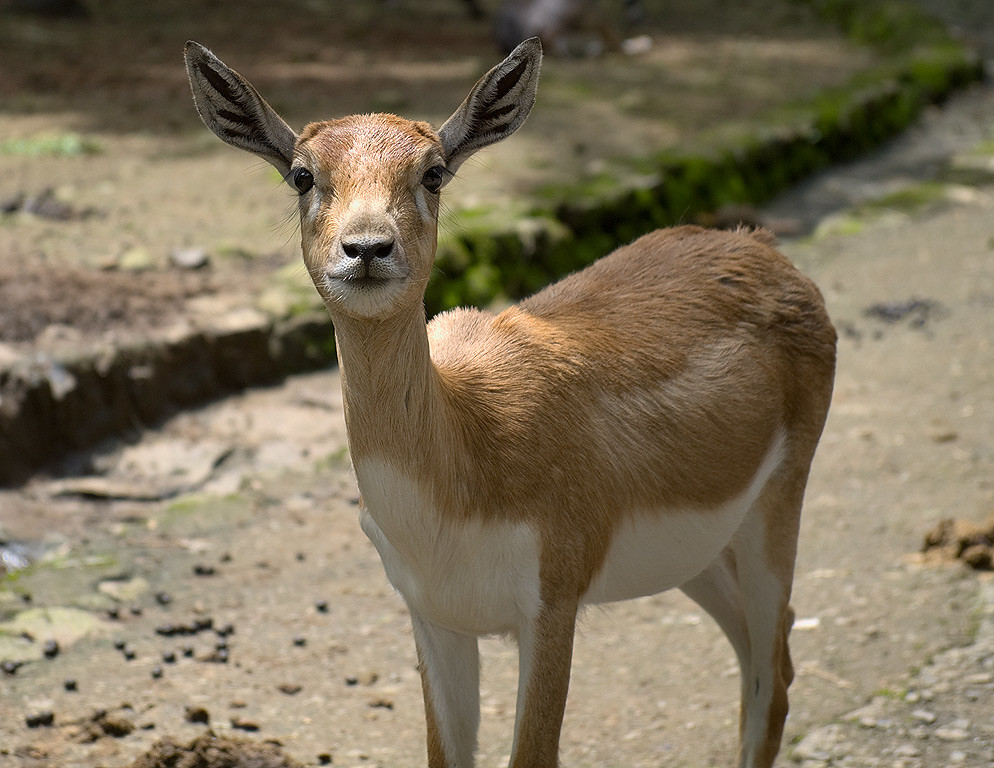The photograph features a juvenile deer standing alertly in the center of a muddy brown path within an enclosure, likely a zoo or sanctuary. The deer, with its delicate brown fur and white underside, gazes directly at the camera with dark, expressive eyes. Its two long, pointy ears, which are gray with black interiors, add to its attentive appearance. The head, neck, and back of the deer exhibit a soft fawn color that transitions into white on the inside of its legs and beneath its belly. The deer stands amidst a mix of brown soil and sparse green grass, indicating a well-maintained, but not overly lush, environment. The scene is highlighted by the deer's delicate features, including a grayish area around its mouth and two flared black nostrils, making it a compelling and endearing portrayal of wildlife within a controlled habitat.